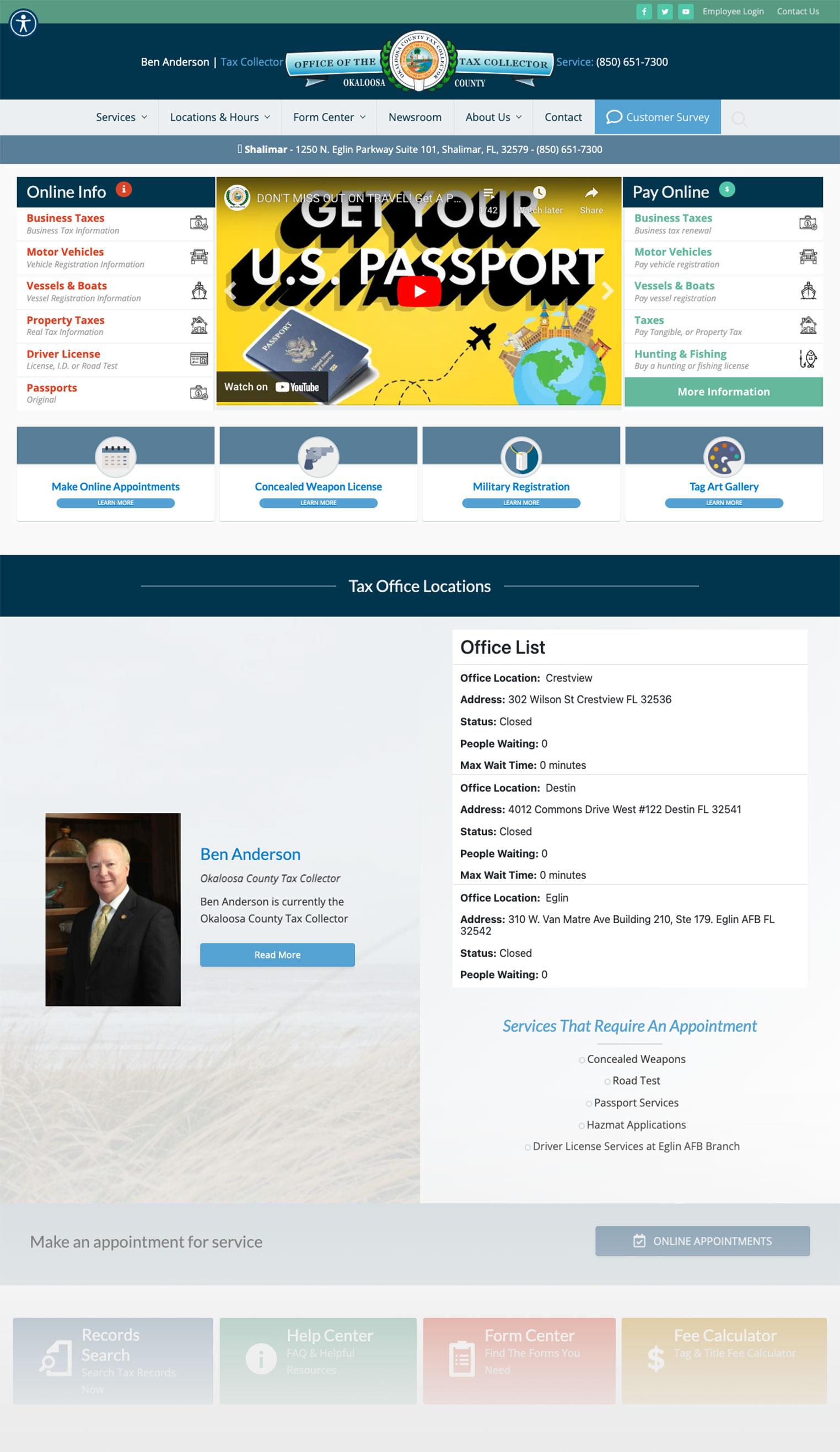A detailed web page for the Ulululu County Tax Collector's Office, somewhere in the United States. The site provides comprehensive information about the various services offered by the office. These services include obtaining US passports, paying property taxes, making online adjustments, registering military tags, and applying for concealed weapon licenses. In addition, the tax collector's office handles motor vehicle registration, vessel and boat registration, and driver's license issuance. The web page also lists the various office locations throughout Ulululu County where residents can access these services. Ben Anderson is the current County Tax Collector, providing a diverse range of services from one central office.